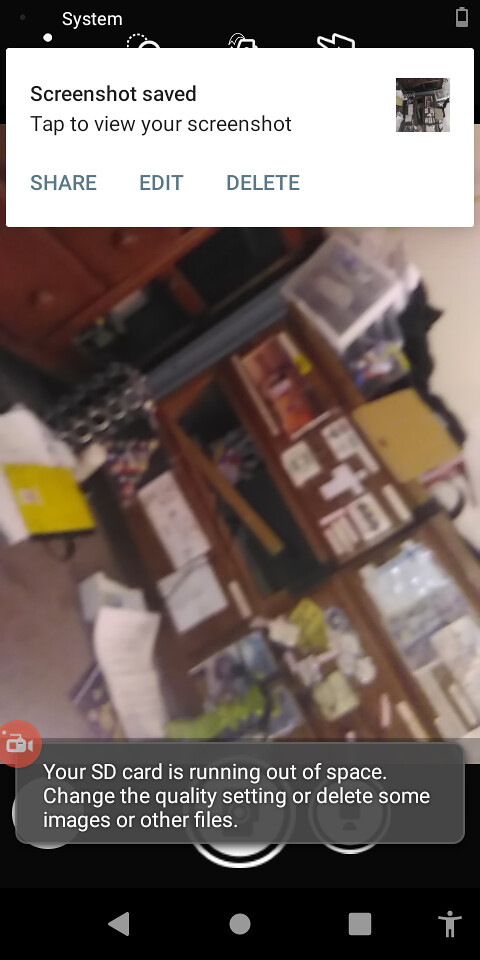A screenshot captured from a cell phone displays a chaotic desk or shelving unit cluttered with an assortment of stickers and scattered papers. The image showcases the disorganization and overwhelm of the space. At the top of the screenshot, a white text bar states "Screenshot saved. Tap to view your screenshot. Share, edit, delete." Additionally, at the bottom of the image, there is a transparent notification bar reading, "Your SD card is running out of space. Change the quality settings or delete some images or other files," overlaid on top of the usual camera buttons.